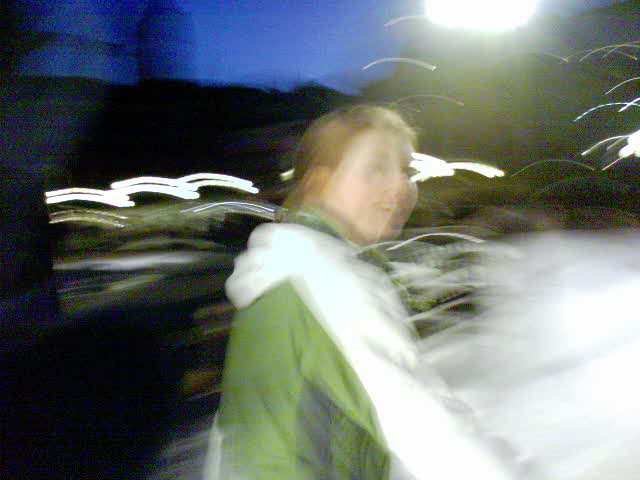In the foreground of this blurred image stands a snowman dressed in a track jacket. The jacket features green at the bottom and white accents extending from the arms and hood. The snowman has white hair, a cheerful smile, and is looking towards the right. The ground around it is blanketed with snow. The background shows blurred lights scattered throughout, with a distinct white light at the top right and a deep blue sky above, transitioning to black towards the back. The scene also includes a series of lights that are blurry and stretch across the screen, creating arcs. Most arcs are white or slightly off-white, with one prominently blue arc. The direction of the blur marks moves from the lower left to the upper right, adding to the dynamic and somewhat chaotic feel of the image. Additionally, there seems to be some kind of bordering or fencing in the background.